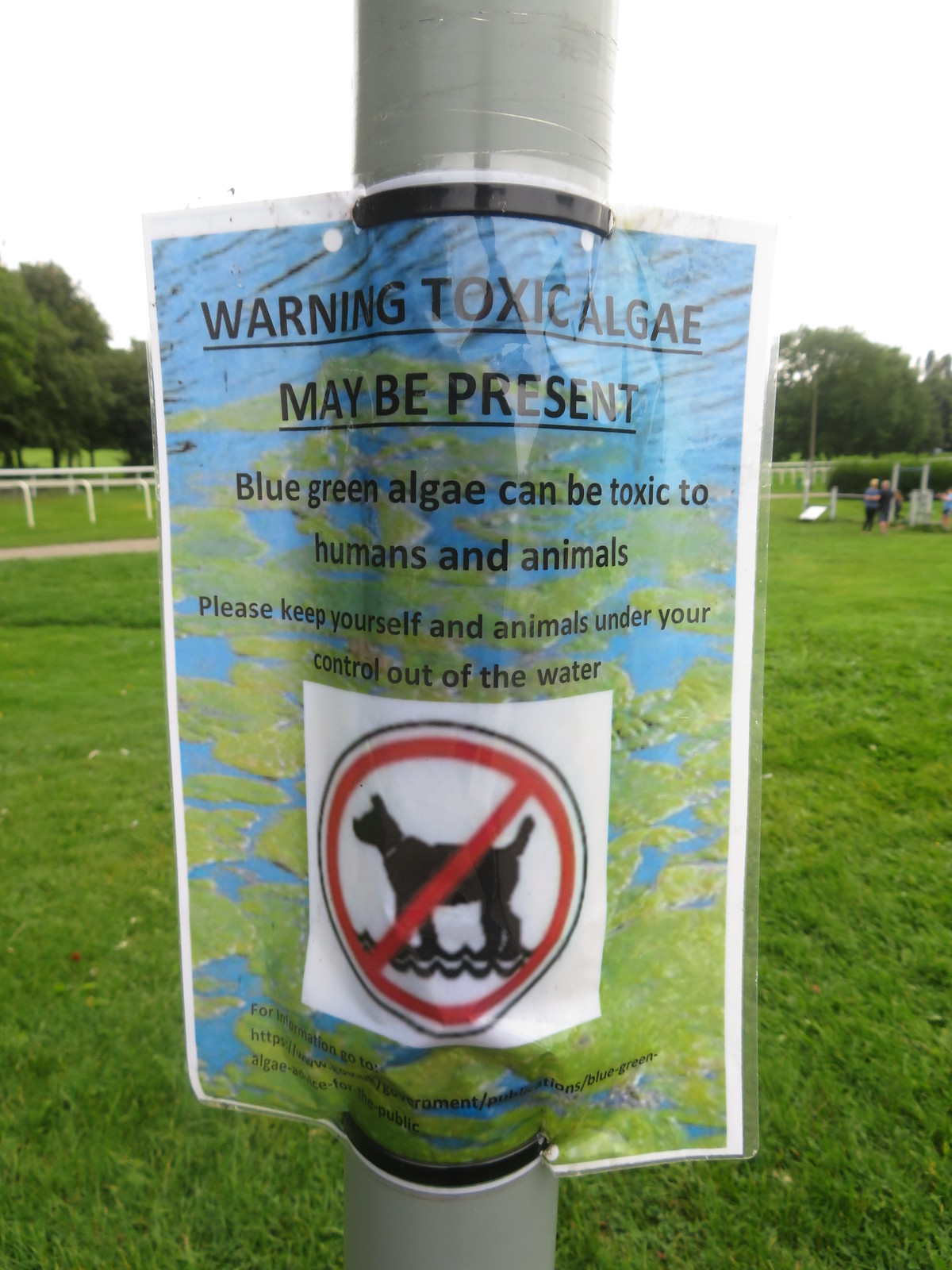The image features a detailed close-up of a warning sign posted on a silver metal pole situated in a grassy field, possibly within a public park. The sign, resembling an 8.5 by 11 inch piece of paper, warns of the presence of toxic blue-green algae in the water. The large black text at the top reads "WARNING: Toxic Algae May Be Present," followed by "Blue-green algae can be toxic to humans and animals" in smaller font, and a cautionary note, "Please keep yourself and animals under your control out of the water." Below this text, there is a graphic depiction of a dog standing in water with a red cross-hatch symbol, indicating that pets should be kept away from the water. The edges of the sign are white while the main background shows an image of a lake with blue and green hues typical of algae. In the background, one can see an expansive grassy area, dotted with trees, and flanked by two white fences. To the right, there are two individuals in the distance. The sky is visible above, suggesting it is daytime, possibly early evening when the sunlight is soft. The overall scene combines elements of green, blue, white, black, red, and gray, painting a vivid reminder to avoid the water where toxic algae may be present. A rectangular object lies at a slant on the ground, although its purpose is unclear.